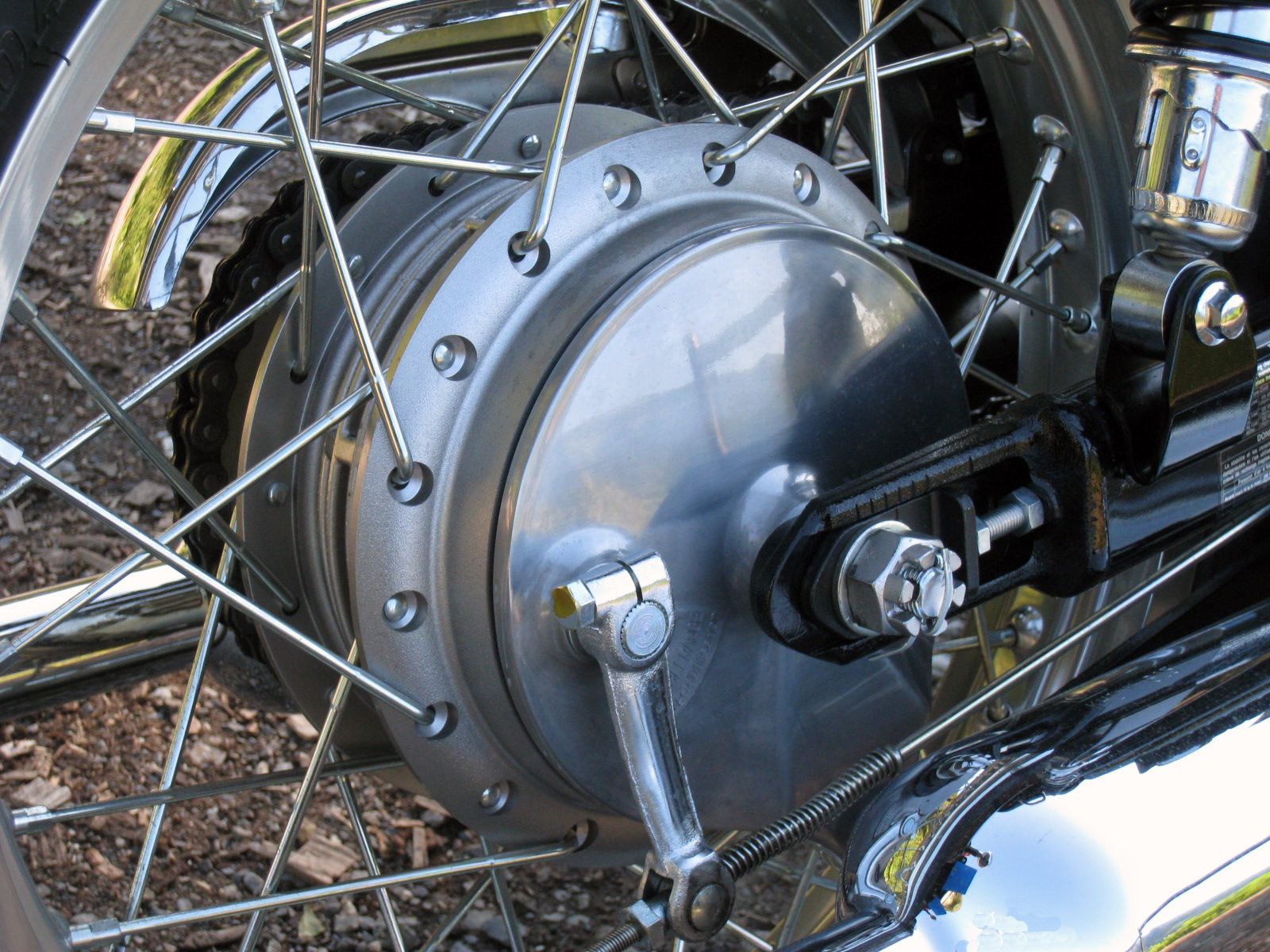This highly detailed, zoomed-in image showcases the intricate mechanics of a motorcycle's rear end. Central to the photograph is a polished silver spoked wheel, with gleaming chrome rods radiating from the solid hub. The image captures the meticulously clean and well-polished components of the bike, including the brake system and the hub of the back tire. To the right, a spring and coil mechanism is visible, suggesting the connection points to other parts of the motorcycle. There's also a hint of a fender on the left side where the chain runs, and the top of a muffler is just visible in the bottom right, adding to the complexity of the image. The almost seamless integration of the grayish outer bearing with the chrome rods highlights the attention to detail in the bike's design. Overall, the picture, taken from the right corner looking towards the left, offers a cross-sectional view of the motorcycle's rear wheel area, emphasizing the sophisticated engineering and polished aesthetics.